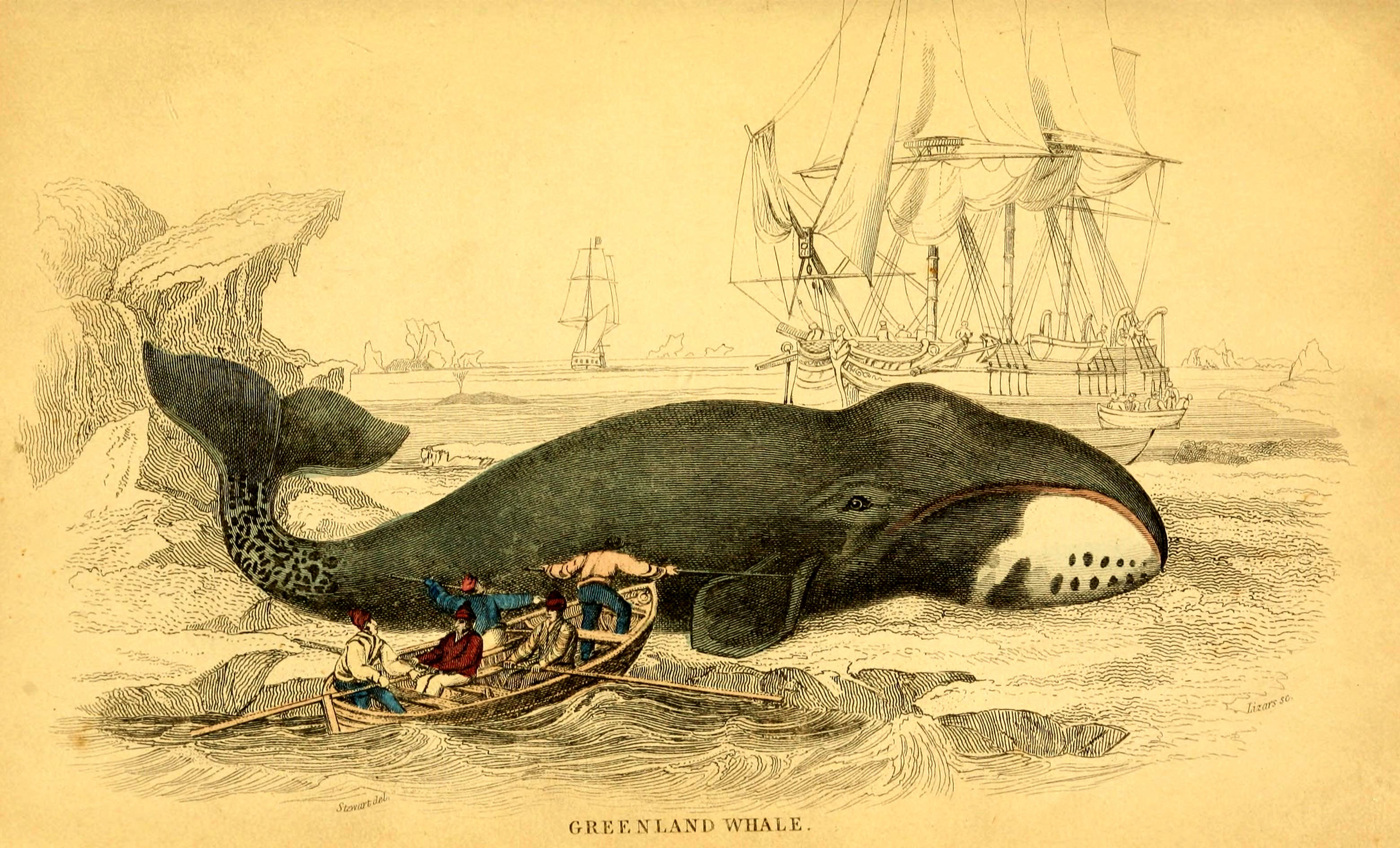This detailed hand-drawn illustration, likely from the 18th century, vividly depicts a scene labeled "Greenland Whale." The illustration appears on sepia-toned paper, suggesting it may have been scanned from an old book or document. At the center of the image is a large whale, primarily black in color, set against a backdrop of yellow hues. The whale is accompanied by a group of sailors in a brown rowboat, numbering between four to five men. These sailors are equipped with oars and are seemingly attempting to harpoon the whale with spears or sticks. The surrounding scene includes ocean waves and several many-masted sailing ships in the background, contributing to the impression of a maritime expedition. The overall illustration, combining black-and-white elements with selective use of color, captures the dramatic and adventurous spirit of historical whale hunts. Though some details, such as whether the whale is beached or at sea, are ambiguous, the artist's detailed portrayal offers a glimpse into the marine life and seafaring endeavors of past centuries.